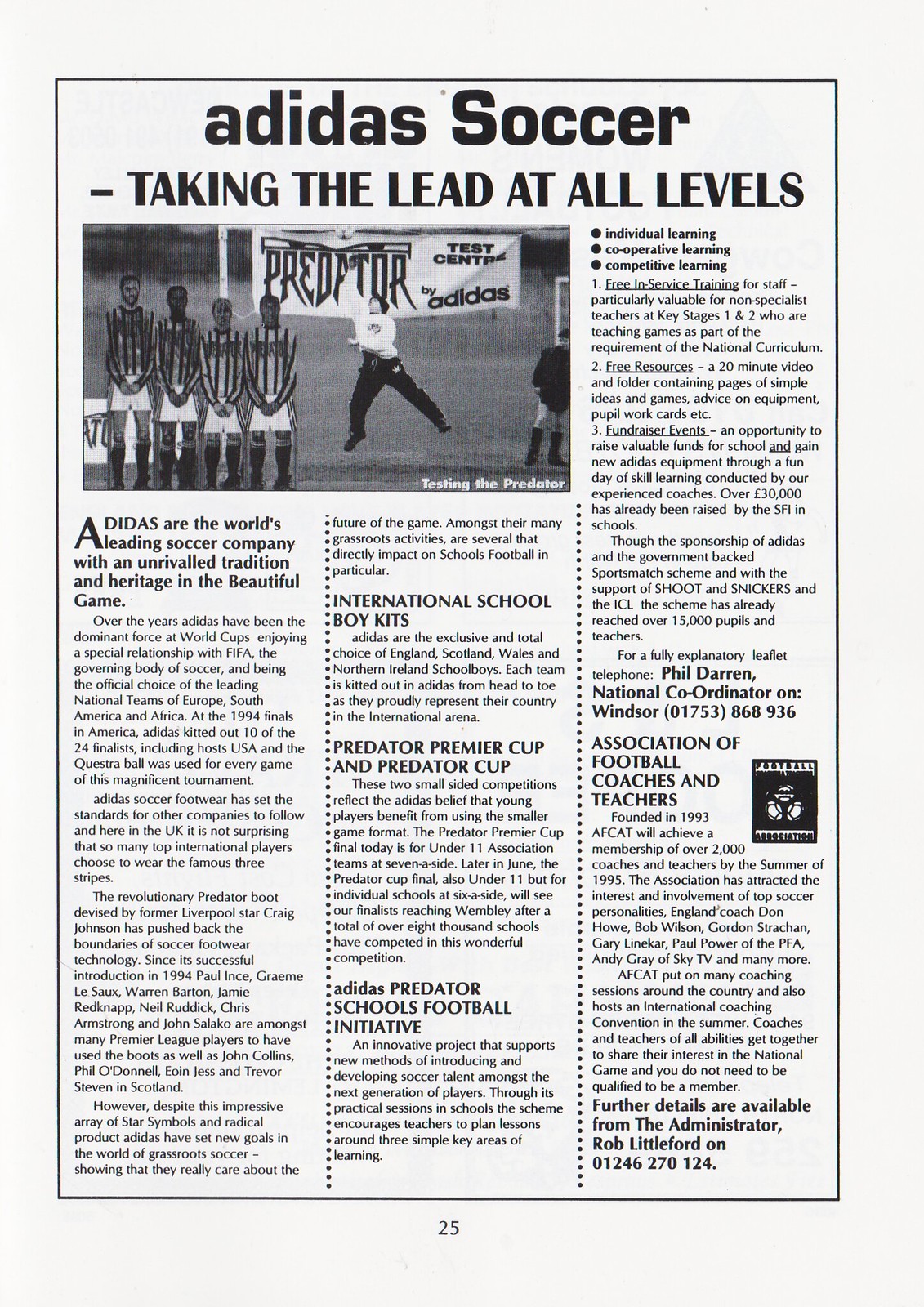This black-and-white newspaper advertisement features the headline "ADIDAS SOCCER: TAKING THE LEAD AT ALL LEVELS" in bold letters. Dominating the page is a striking photograph of four soccer players in striped jerseys and white shorts, standing in formation. Behind them, a goalie clad in a white jersey and black pants is seen leaping impressively, attempting to intercept a soccer ball.

The accompanying text celebrates Adidas as the world's leading soccer company, praising its rich tradition and heritage in the sport. It highlights Adidas' long-standing relationship with FIFA and its dominance in international tournaments, including its significant presence in the 1994 World Cup. The advertisement underscores the brand's commitment not only to professional soccer but also to grassroots initiatives, mentioning various programs like the Predator Premier Cup and the Predator Cup. These competitions aim to develop young talent through smaller-sided games. Additionally, it notes the Adidas Predator School Football Initiative, which provides resources and training for schools, benefiting over 15,000 pupils and teachers.

The page also references the Association of Football Coaches and Teachers (AFCAT) established in 1993, promoting its efforts to support soccer coaching across the UK. The ad showcases Adidas' dedication to fostering the next generation of soccer players and educators, ensuring that the sport's future remains bright.